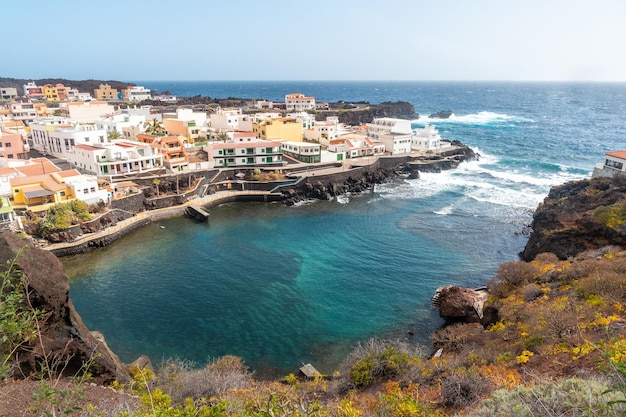This high-angle shot captures a picturesque seaside town nestled around a small, turquoise cove. The town, with an old-world charm, appears to be European or South American in origin rather than American. The ocean, a vibrant blue, forms a background to the scene, and the waves crash turbulently at the entrance to the harbor.

On the left side of the image, a dense urban area featuring hotels, apartments, and multi-story buildings in colors of white, yellow, and light peach is perched atop dark brown rocky cliffs. These buildings stretch upwards and right next to the cliff edges, giving an almost island-like appearance. 

The cove itself is U-shaped and cradled between two rocky ridges. The right-hand side is characterized by a rugged, brown, rocky surface topped with varied vegetation, including tan bushes, vibrant yellow flowers, and green shrubbery. In contrast, the left side of the cove has a densely built urban area with tall buildings almost reaching the cliff's edge. The water is a mix of teal and dark blue, with white-capped waves adding dynamic energy to this tranquil yet vibrant coastal setting.